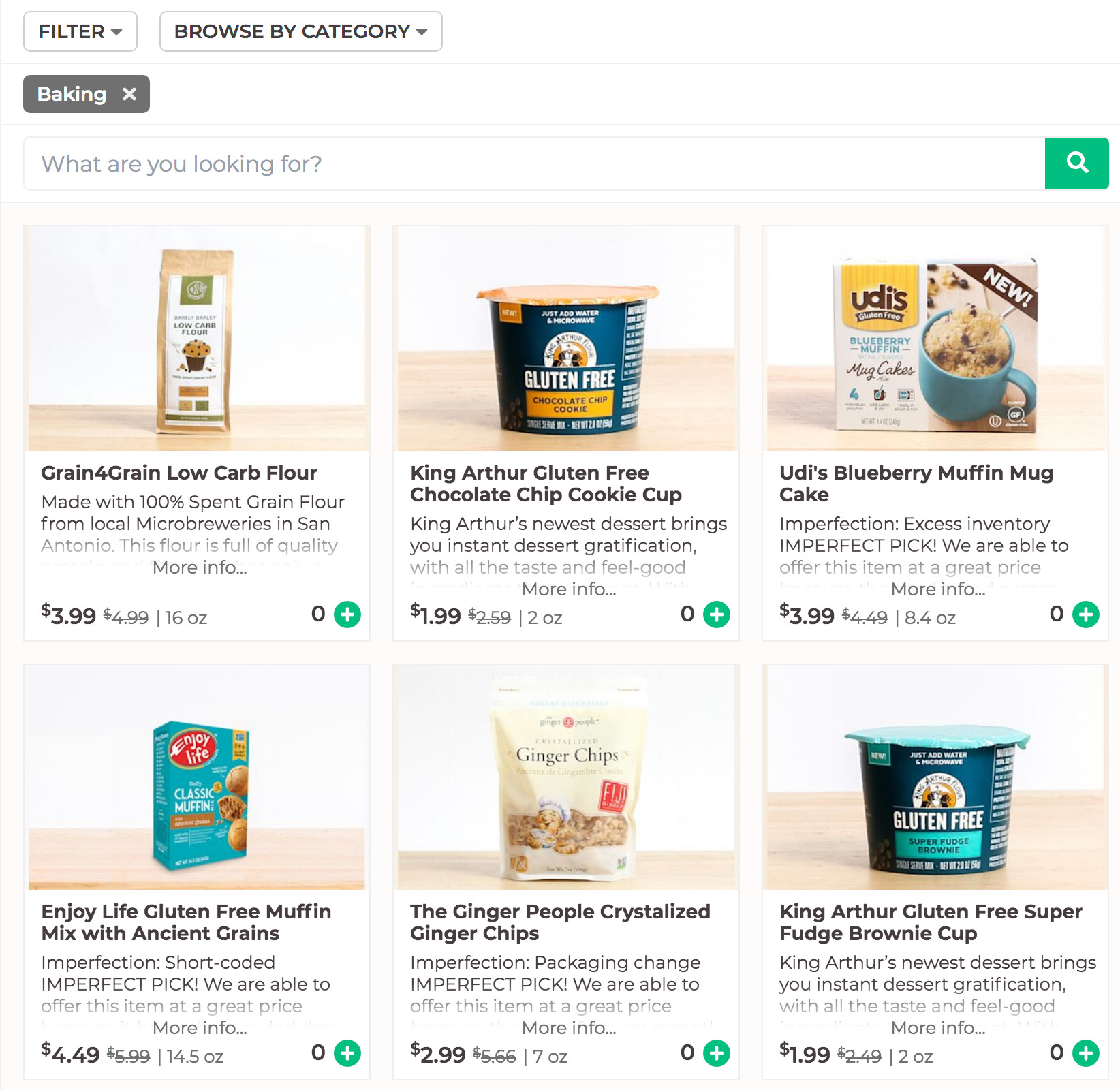The image features a user interface with a white background, prominently displaying various food items and filters. At the top, there are two dark gray rectangles. The first rectangle contains the text "Filter" and "Browse by Category," while the second rectangle, in light gray, says "Bacon" with an "X" next to it, indicating a selected filter. Below these, another light gray rectangle contains the text "What are you looking for?" next to a green search icon featuring a white magnifying glass.

The main section of the image is divided into two rows, each with three featured food items. The first row includes:
1. A product labeled "Grain for Grain, Low-Carb Flour" alongside an image of cookies. 
2. Another labeled "King Arthur Gluten-Free Chocolate Chip Cookie," depicted as a chocolate chip cookie in a cup.
3. "Udi's Blueberry Muffin Mug Cake," shown as a chocolate mug dessert.

The second row features:
1. "Enjoy Life Gluten-Free Muffin Mix with Ancient Grains," with an accompanying image.
2. "The Ginger People Crystallized Ginger Chips."
3. "King Arthur Gluten-Free Super Fresh Brownie Cookie."

Beneath each product, its respective price is listed: $3.99, $1.99, and $3.99 for the first row, followed by $4.49, $2.99, and $1.99 for the second row. All items are noted to be on sale. The products are displayed on a white and beige surface, which could be a table or possibly a mock-up due to the zoomed-in nature of the image.